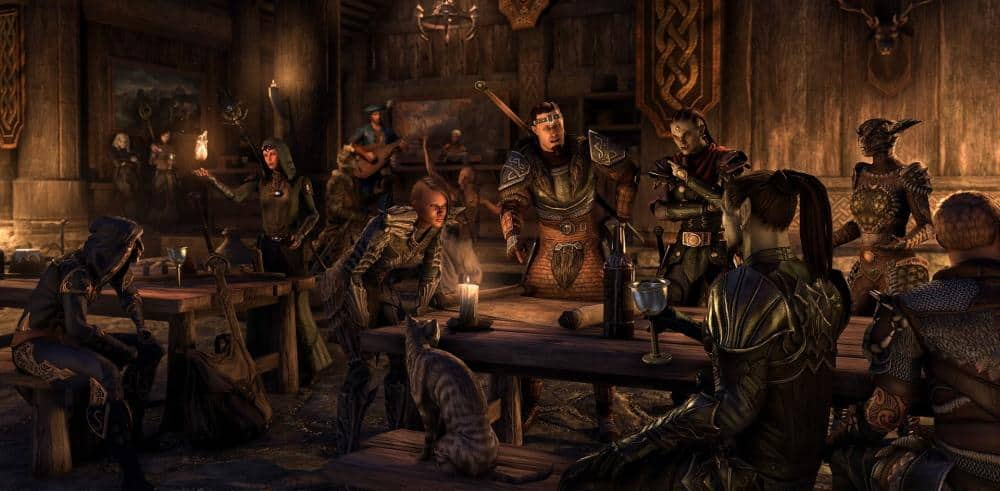The computer-generated image features a diverse assembly of characters from the Elder Scrolls series, particularly from the Elder Scrolls Online. At the forefront, a variety of races, including elves with pointed ears, lizard-like Argonians, and humans, are gathered around a long, horizontal wooden table. Some characters hold goblets or wine glasses, suggesting a communal gathering in what appears to be a medieval pub setting. The image captures a dimly lit room, illuminated primarily by candles. Adding to the fantasy ambiance, one character on the left side of the image is conjuring a flame above their hand. The characters are clad in thick, dark armor, primarily silver but rusted, indicating well-worn equipment. Many of these armored individuals have swords either sheathed on their backs or propped against the table. An ordinary gray house cat sits beside the characters, adding a touch of whimsy. In the background, more people can be seen, including a woman engaged in conversation. Mounted on the brown, wooden walls are dead deer heads, enhancing the medieval atmosphere. The group appears to be engaged in an important discussion, emphasizing the significance of the gathering.